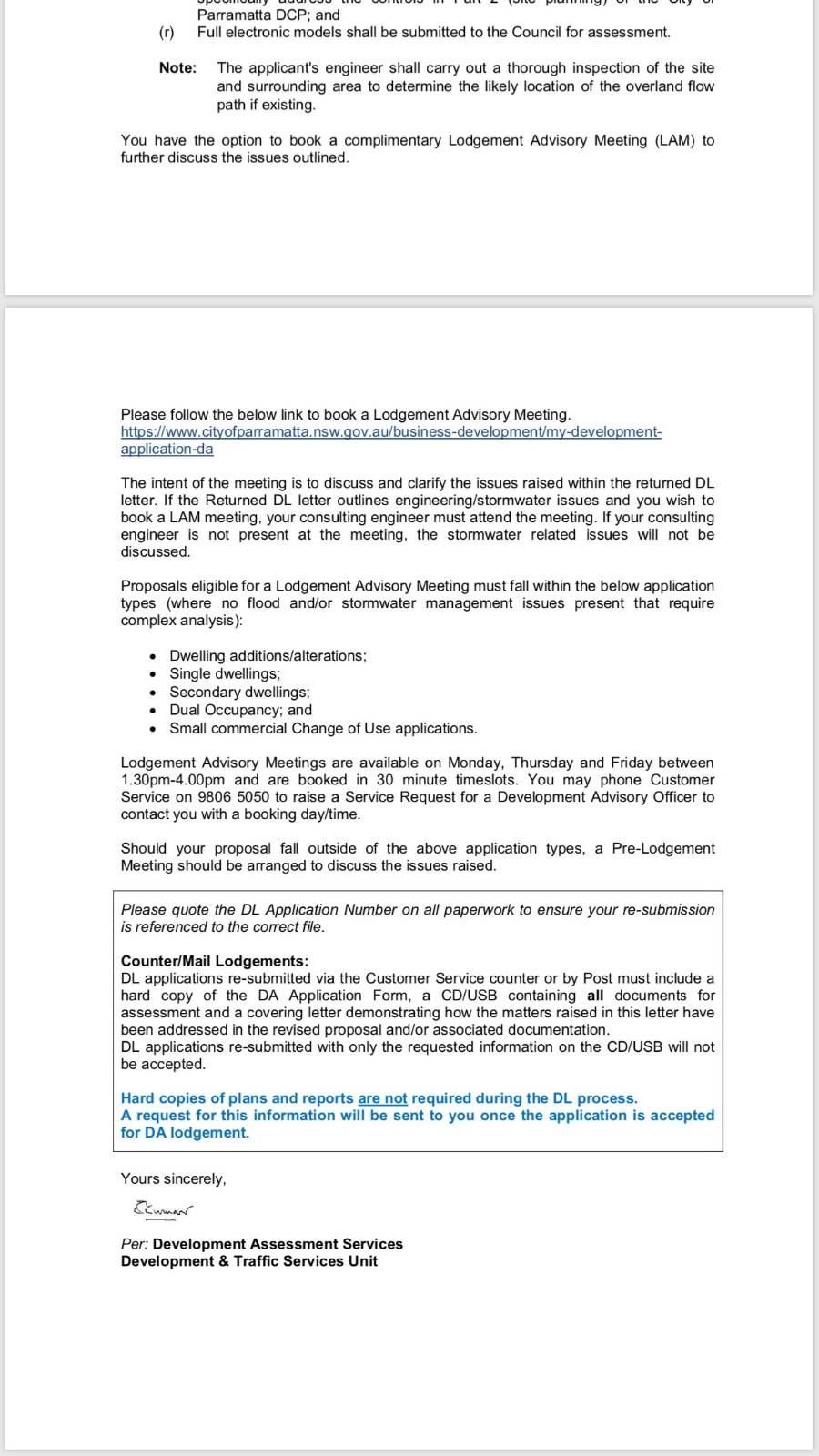Detailed caption: 

The image shows a detailed document from the City of Parramatta Council regarding business development procedures. The top portion of the first page is partially cut off, displaying only the bottom third. This section references the "Parramatta DCP" and emphasizes the submission of a full electronic model to the Council for assessment. It includes a note advising that applicants and engineers should conduct a thorough inspection of the site and surrounding area to identify potential overland flow paths.

The document offers the option to book a complimentary lodgement advisory meeting (L-A-M) to discuss matters in more detail. Instructions on how to book such a meeting are provided, including a hyperlink. The advisory meetings are intended to discuss and clarify issues raised by the return D-L letter and are available on Mondays, Thursdays, and Fridays from 1:30 PM to 4:00 PM, in 30-minute time slots.

A prominent box on the page asks applicants to quote their D-L application number and include all relevant paperwork to ensure correct resubmission referencing. It also states that hard copies of plans and reports must be submitted for resubmissions done via the customer service counter or by post. Additionally, hard copies are required during the D-L process and requests for such information will be sent out once the application is accepted.

The document concludes with a formal closure, "Yours sincerely," signed by the Development Assessment Services.